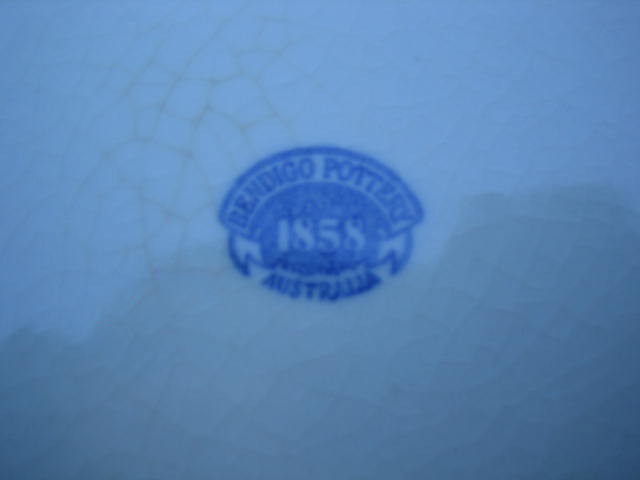The image depicts a very close-up, poor-quality photograph of a cracked ceramic piece, likely the bottom of a piece of pottery, where a stamp has been applied. The stamp appears in blue and is somewhat legible despite the shadows casting across the surface. The stamp reads "Bendigo Pottery 1858 Australia," with "Bendigo Pottery" forming an arc at the top, "1858" in the oval-shaped middle section, and "Australia" at the bottom. The ceramic surface is primarily white with a blue background where the stamp sits. The image shows distinct lines and geometric crackle patterns, particularly noticeable in the upper left corner. The close-up nature of the photograph renders some details blurry, but the stamp's content is clear enough to be read.